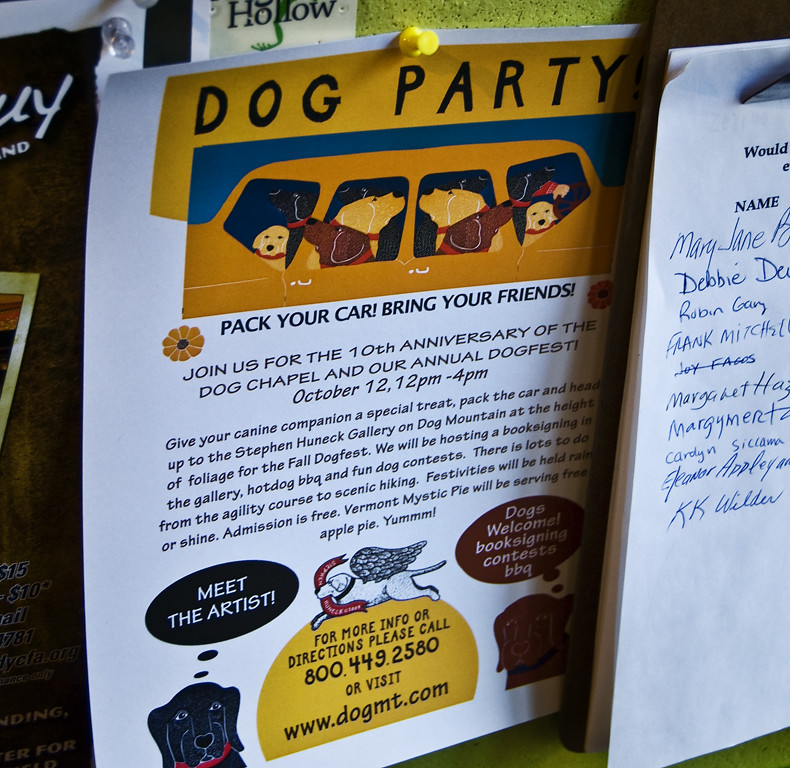The photo shows a square-shaped bulletin board located in a communal area, with a primary focus on a single attention-grabbing post held up by a yellow thumbtack at its center. The featured paper, appearing to be printed at home, prominently announces a "Dog Party" in a vibrant orange heading. The upper portion of the paper showcases illustrations of dogs, resembling golden retrievers, seated in an orange car, evoking a cartoonish charm.

Beneath the illustrations, the text invites the community to, "Pack your car, bring your friends. Join us for the 10th anniversary of the Dog Chapel and our annual dog fest," scheduled for October 12th, from 12 p.m. to 4 p.m. Below this invitation, a detailed paragraph entices attendees to treat their companions and head to the Stephen Hunick Gallery on Dog Mountain. Additional information bubbles across the bottom, announcing various activities like meeting the artist, contests, hot dogs, and a barbecue, with a note indicating that dogs are welcome.

A yellow circular bubble on the bottom left corner provides further details, stating, "For more info or directions, please call 800-449-2580 or visit www.dogmt.com," accompanied by an illustration of a winged dog, affectionately known as the angel dog. To the right side, there's another paper with handwritten names in blue ink, suggesting a sign-up sheet. A dark blue cloth piece, held by a clear thumbtack, and a smaller paper with "hollow" written on it are also pinned nearby.